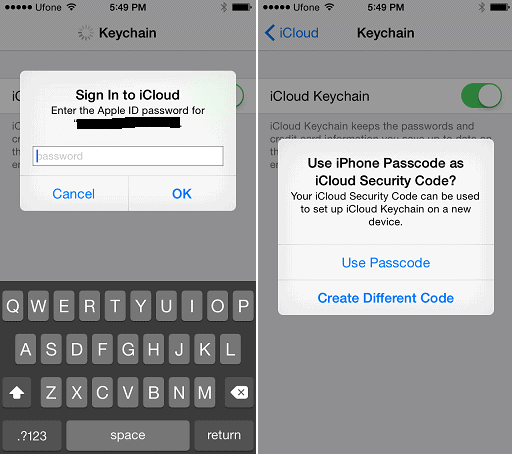The image features two cell phone screens displayed side-by-side, each in a tall rectangular format against a gray, grayed-out background. Each screen has a pop-up window with different content.

**Left Screen:**
- **Pop-Up Window:** The light gray pop-up asks the user to "Sign into iCloud: Enter the Apple ID password for," with the text following "for" blacked out. 
- **Password Field:** A white rectangular input box labeled with the faint word "password" and a blue cursor blinking on the left side of it.
- **Buttons:** Two blue buttons labeled "Cancel" on the left and "OK" on the right beneath the password field.
- **Additional Screen Details:** On the gray background above the pop-up, the time is displayed as 5:49 PM, and the word "Keychain" is visible. Below the pop-up, the cell phone keyboard is partially visible.

**Right Screen:**
- **Pop-Up Window:** The light gray pop-up inquires, "Use iPhone passcode as iCloud security code?" followed by the information: "Your iCloud security code can be used to set up iCloud Keychain on a new device."
- **Buttons:** Two blue buttons stacked vertically, the top one reading "Use Passcode" and the bottom one reading "Create Different Code."
- **Additional Screen Details:** Similar to the left screen, the time displayed is 5:49 PM. The grayed-out part of the screen shows "iCloud" in blue, "Keychain," and an activated green toggle switch next to the words "iCloud Keychain."

The overall layout and content of the image provide a clear presentation of the prompts and options faced by the user when dealing with iCloud and Keychain settings on their devices.